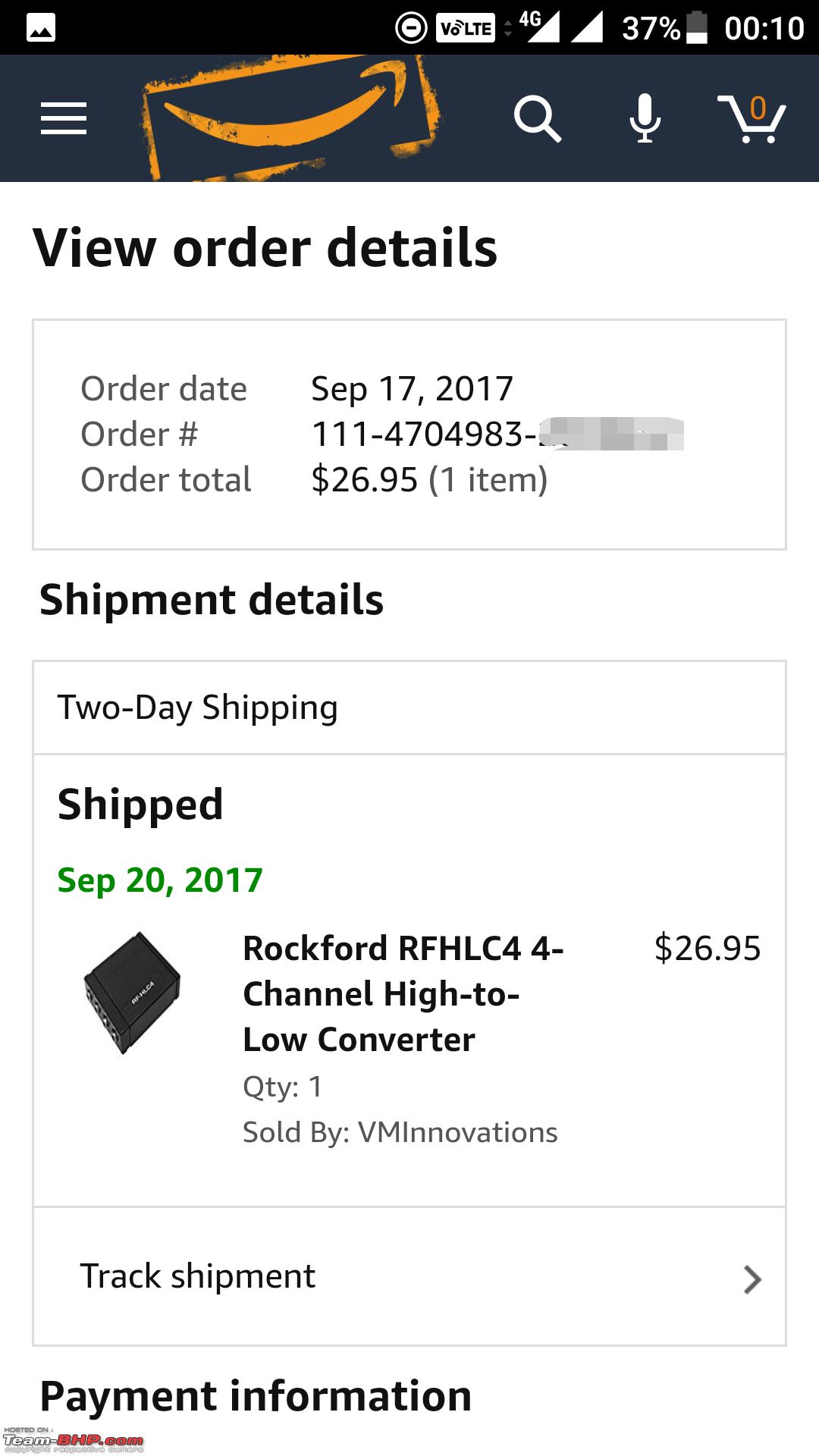This mobile screenshot displays the 'View Order Details' page on Amazon.com. At the top, prominently situated on the left, is the familiar Amazon.com logo. Adjacent to it, to the right, is the Prime logo depicted as a yellow arrow within a yellow box, and a menu icon is located to its left. To the right of the Prime logo, a set of icons represents the search functionality: a magnifying glass, a microphone, and a shopping cart icon, all aligned alongside a blue banner.

Just below this header section, the page title "View Order Details" is prominently displayed in large black letters on a white background. Underneath this title, a thin, outlined gray box provides essential order information such as order date, order number (with a portion edited out), and the total amount.

Following this, the page titles 'Shipment Details' in bold black letters. Directly beneath, a section specifies the shipping method as 'Two Day Shipping', highlighting 'Shipped September 20th, 2017' in green. Adjacent to this text is a thumbnail image of the product, accompanied by a brief product description on its right. To the far right of this box, the total amount for the order, $26.95, is clearly stated.

The bottom section features the option 'Track Shipment' with an arrow pointing to the right, suggesting further action. Beneath this, a section labeled 'Payment Information' is visible, although the specific details have been edited out of the screenshot.